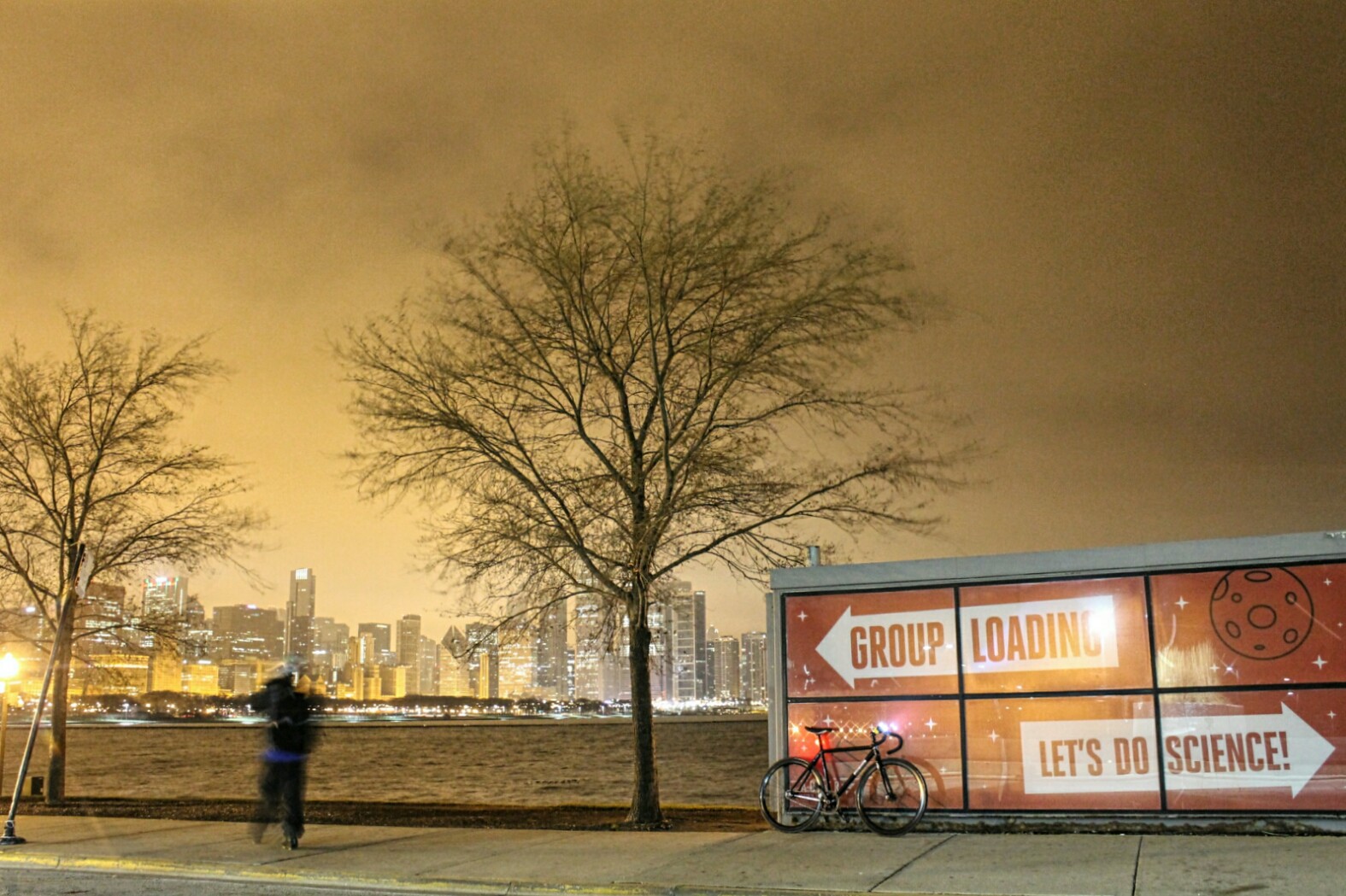This photograph captures an atmospheric scene either in the early morning or late evening, characterized by a yellow, dusky sky tinged with either fog or smoke. In the distant background stretches the illuminated cityscape with tall buildings, extending from the left to just past the middle of the frame. The foreground reveals a detailed urban setting: a blurry figure, likely male, clad in dark clothing including black pants, a blue shirt, and a black backpack, walking along a sidewalk. 

Two bare trees devoid of leaves frame the scene on the left, their myriad branches spreading out. Leaning against a prominent signpost that partially obstructs the city view is a black ten-speed bicycle. The sign, predominantly red, features two white arrows with the upper arrow pointing left labeled "Group Loading" and the lower arrow pointing right labeled "Let's Do Science." Next to this sign is a gray advertising display case with an advertisement featuring an orange background and an illustrated planet in the upper right corner. In the background, below the cityscape, the terrain could be interpreted as either a grassy field or a body of water like a lake, adding an additional layer of depth to this beautiful urban scene.